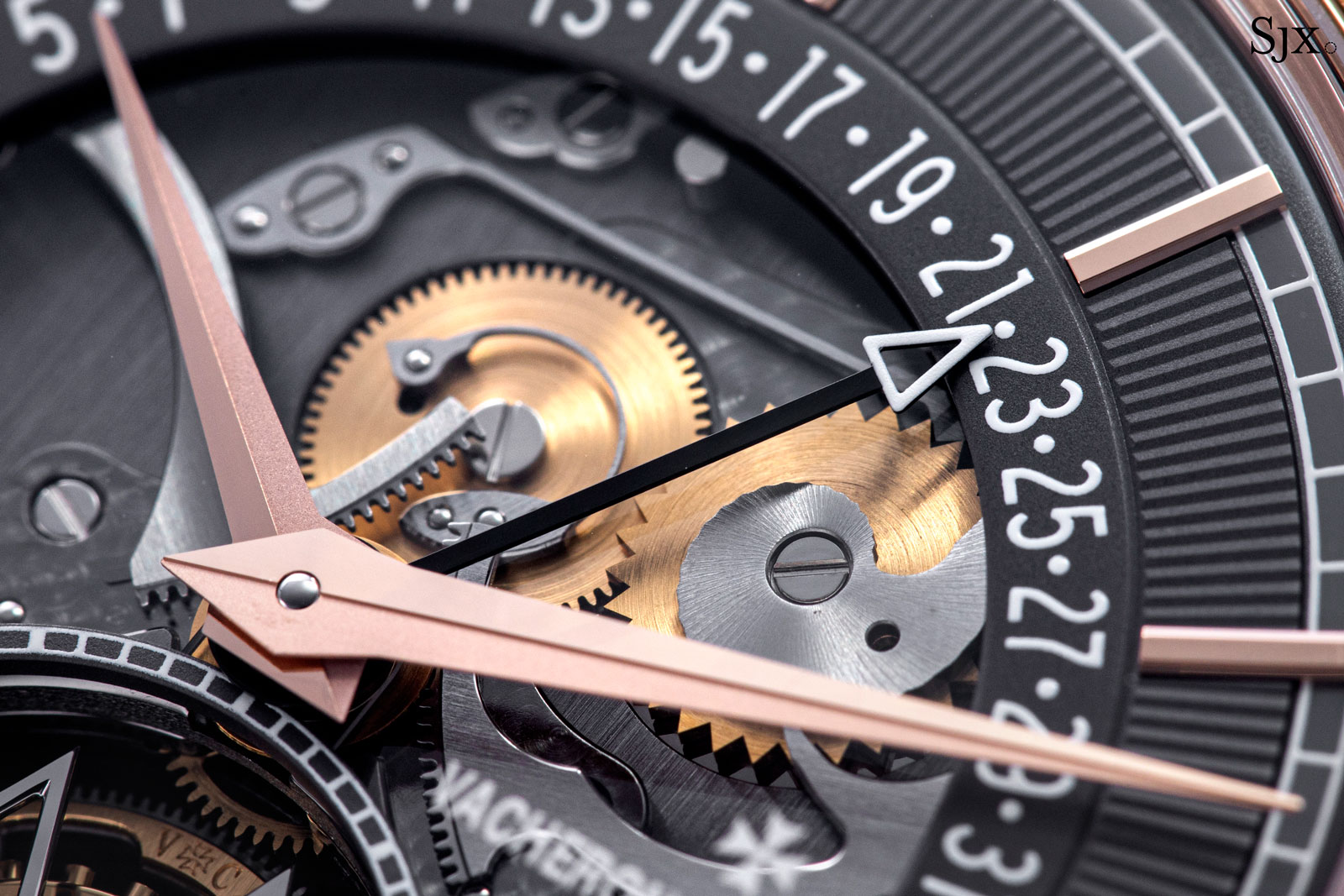The image is a detailed close-up photograph of a watch’s inner workings, with the clock face partially visible. The overall shape of the photo is rectangular, and the watch's face occupies most of the scene. The watch mechanism showcases intricate golden and silver gears and cogs, meticulously arranged and visible through a transparent section of the watch. The rim is rose gold, giving the piece a luxurious feel.

Notably, the watch displays three hands: the hour and minute hands are rose gold, while the second hand is distinct with a black color and a white arrowhead. The time appears to be around 10:15, with the second hand pointing at 22 seconds.

The watch features a number sequence painted in white along the inner edge of the face, progressing from 15 to 31 in odd numbers. Additional details include black text reading "SJX" in the top right corner and partially visible text “V-A-C-H-E-R,” indicating some form of branding. The outer edge of the face is gray, adding contrast and depth to the intricately designed timepiece.